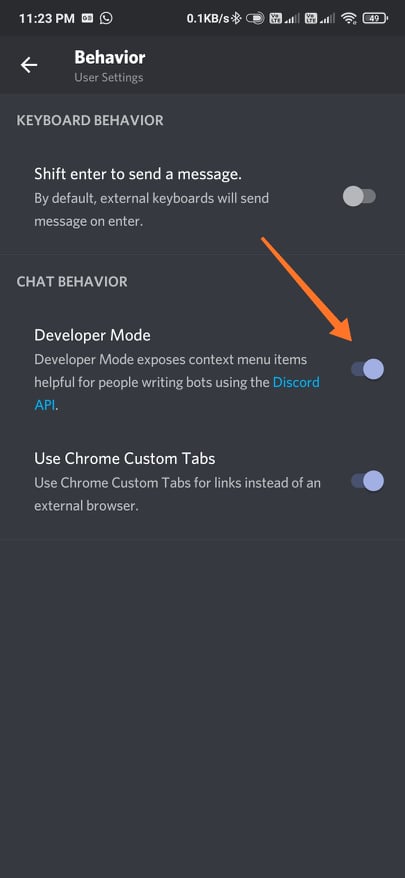A screenshot captured from a mobile device displays a section of the "Behavior User Settings" on the screen. The top of the interface features a black bar with white text labeled "Behavior User Settings," and an arrow pointing left for navigation. Below that, the heading "Keyboard Behavior" indicates an option labeled "Shift-Enter to send a message," with an explanation that external keyboards will default to sending messages via the Enter key unless toggled otherwise. A toggle switch is available to enable or disable this feature. 

Further down, under "Chat Behavior," there's an option for "Developer Mode," which is described as a feature that reveals content menu items useful for those writing bots utilizing the Discord API. This option also has an associated toggle switch. 

The last section addresses the use of "Chrome Custom Tabs," explaining that this setting allows links to be opened using Chrome Custom Tabs instead of an external browser, and it too contains a toggle switch for user convenience.

An orange arrow highlights the toggle switch beside the "Developer Mode" option, indicating that the person who took the screenshot is drawing attention to this setting, likely to suggest enabling or disabling it based on specific needs.

The status bar at the top of the screen shows the time as 11:23 p.m., alongside two app notification icons. Additional indicators include the battery life, Wi-Fi signal strength, and the cellular signal bars.